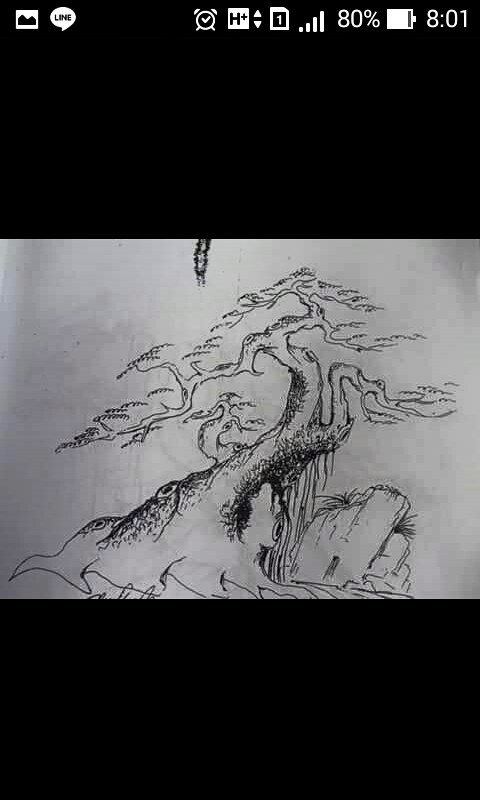This image is a detailed charcoal and ink or pencil sketch displayed on the screen of a cell phone or tablet. It is framed by a solid black background, with a standard white paper background for the artwork itself. The top of the screen shows various white icons indicating the device's status: the time reads 8:01, the battery is at 80%, and full Wi-Fi signal bars are visible. There is also a speech bubble notification, a box with a number one, and several other icons including one labeled M+.

The sketch features a barren, intricate tree with winding, ethereal branches that tend to slope low to the ground, evoking a somewhat fantastical or spooky atmosphere. Its broad, gnarly trunk extends upwards with visible roots, and its branches twist in multiple directions. Notably, the tree appears on the edge of a cliff or mountain by the ocean. To the right of the tree, elements such as a tall rock with plants and a dark, shaded area under the right-most branch add depth and texture to the scene. Below the tree, a cylindrical piece is visible, hanging downwards. The overall composition of the branches and surrounding landscape enhances the spectral quality of the artwork.